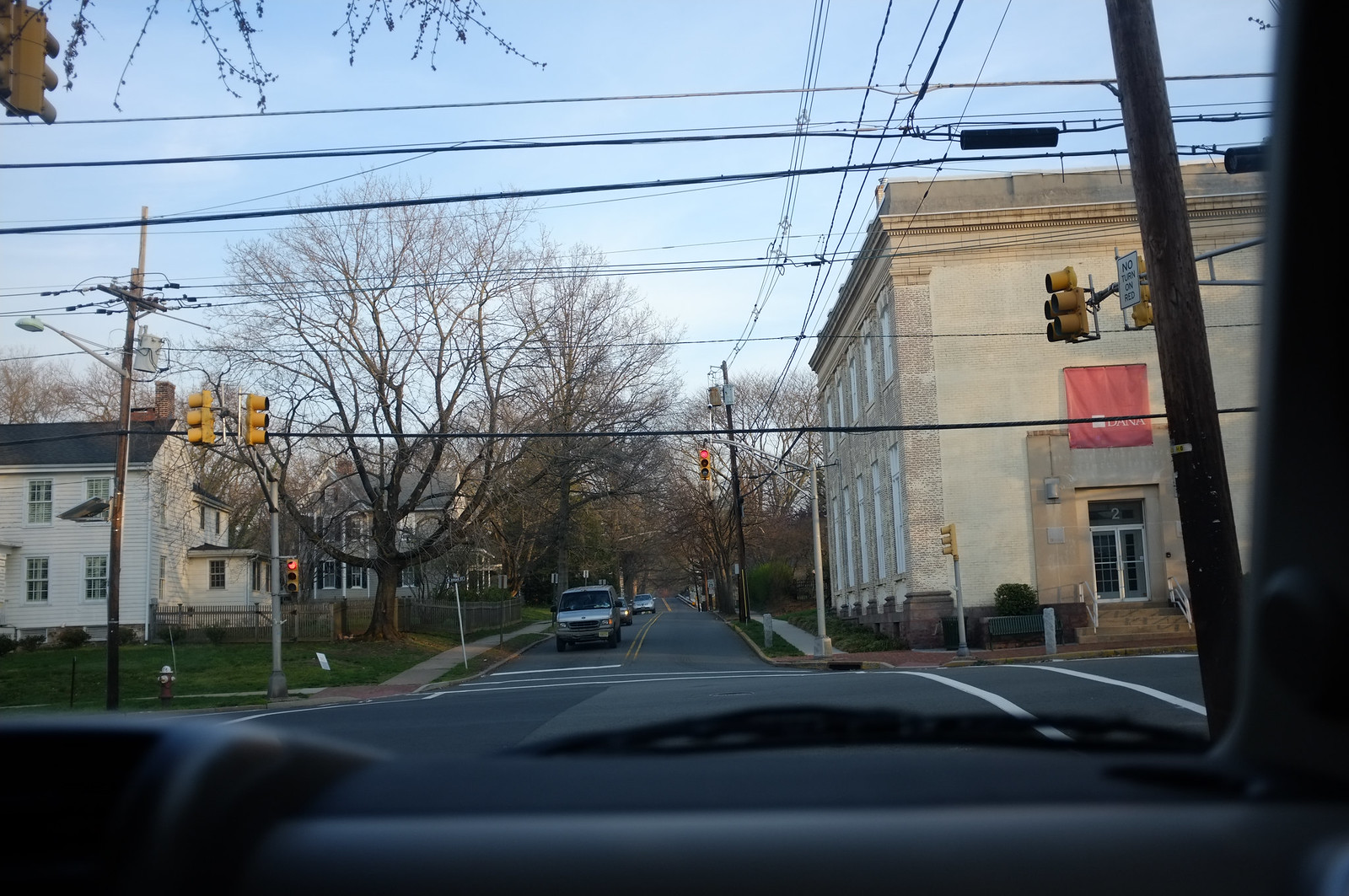A view through the windshield of a car reveals a slightly winding road made of black asphalt, adorned with white lane markings. The car's black dashboard frames the scene, giving a sense of perspective. On either side of the road stand light brown and cream-colored stone tile buildings, their earthy tones contrasting with the bare, leafless trees that line the street. Power lines run parallel to the road and span overhead, completing this urban landscape.